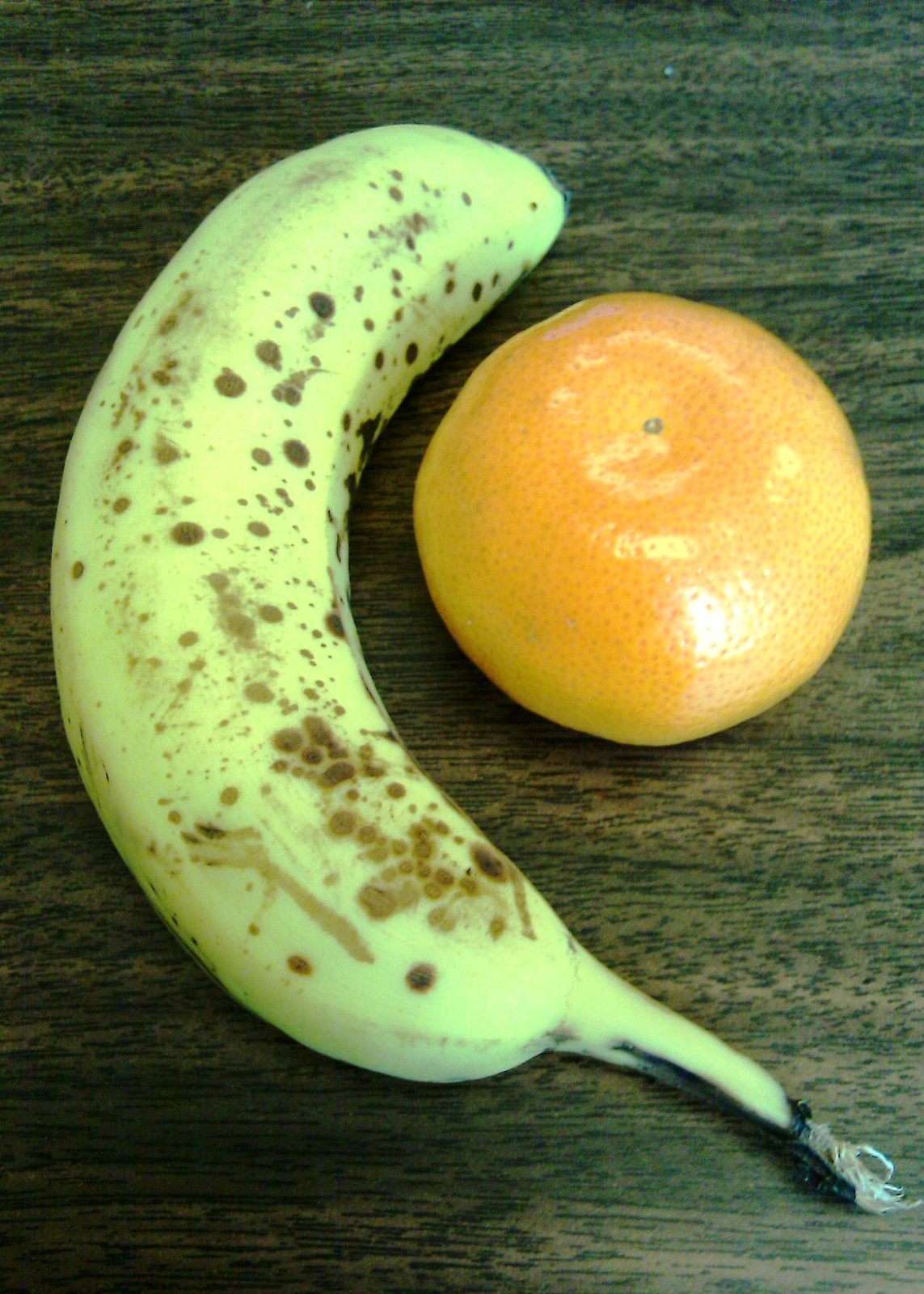A vibrant, detailed image captures a ripe banana and a shiny orange lying next to each other on a dark wooden table. The banana, positioned on the left, features a yellow peel speckled with numerous small brown spots, indicative of its ripe state. Its long stem sits at the bottom of the picture. Nestled comfortably in the curve of the banana is the orange, located on the right side of the frame. The orange appears almost unnaturally shiny, giving it a plastic-like appearance, yet it is small and perfectly round with a tiny remnant of the stem at the top. The juxtaposition of the fruit highlights their contrasting textures and colors, with the orange taking up about half the length of the banana. Both fruits remain unopened, emphasizing their unblemished and natural forms.